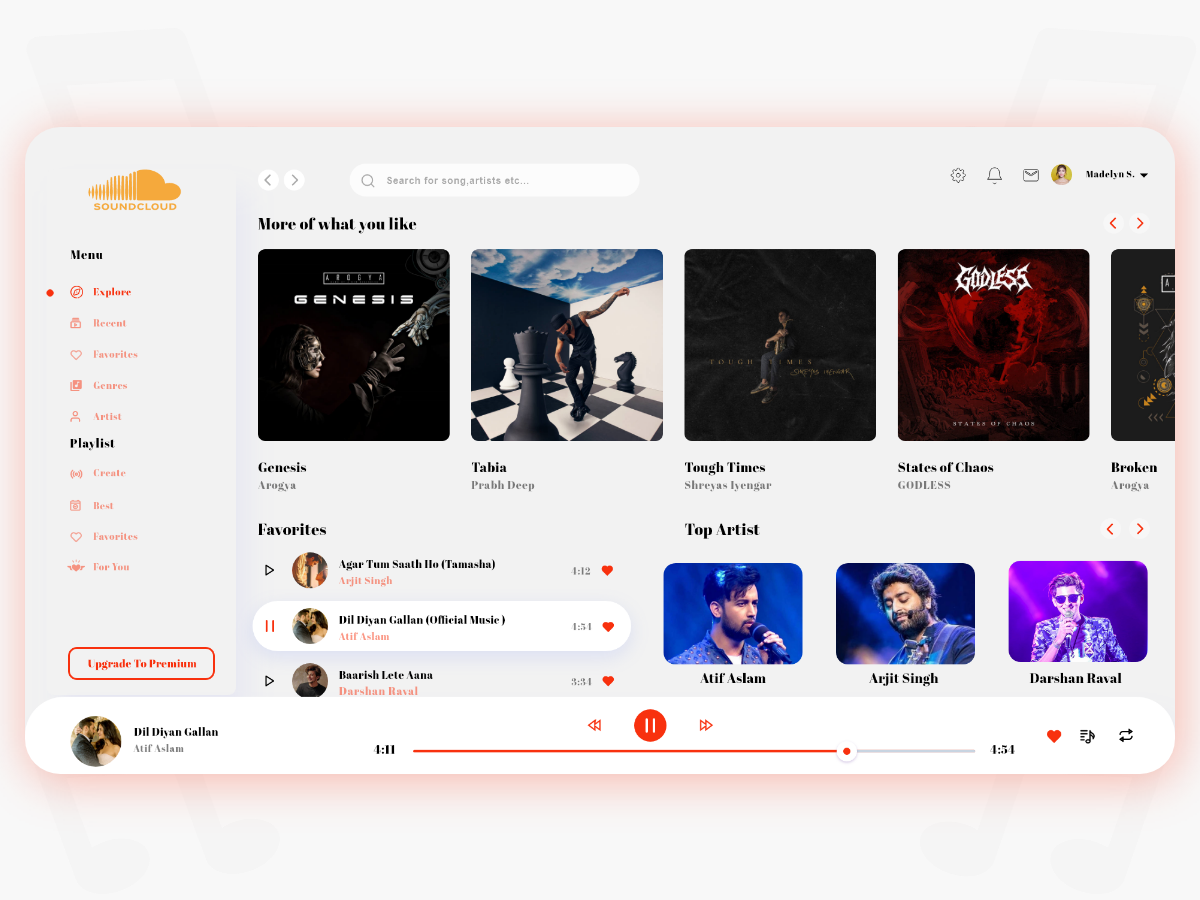The image is a screenshot of a SoundCloud interface displayed on a computer screen. The overall design features a white central area bordered by a vibrant pink background. In the upper left corner of the screen, the iconic orange SoundCloud logo is visible, resembling a cloud. Beneath the logo is a vertical menu containing several options: "Explore," "Renewal," "Favorites," "Genres," and "Artist."

Below this list, there is a section titled "Playlist," which includes options such as "Create," "Best," "Favorites," and "For You." At the bottom of the menu bar, there is a prominent "Upgrade to Premium" button.

On the right side of the interface, at the top, there is a search bar followed by several icons: a gear icon for settings, a bell icon for notifications, a mail icon, and a drop-down menu for the user account, which belongs to a person named Madeline. Below these icons, the heading "More of What You Like" is featured, followed by a series of album covers including titles like "Genesis," "Tabla," "Tough Times," "States of Chaos," and "Broken."

Further down, the screenshot displays the "Favorites" section with corresponding content and, to its right, the "Top Artist" section. At the very bottom of the screen, there is a red progress bar indicating the playback of a song. Control buttons for navigating the track are present: back, forward, and pause. The currently playing song appears to be titled "Dill, Dylan, Gollin," and judging by the progress bar, the listener is more than halfway through the track.